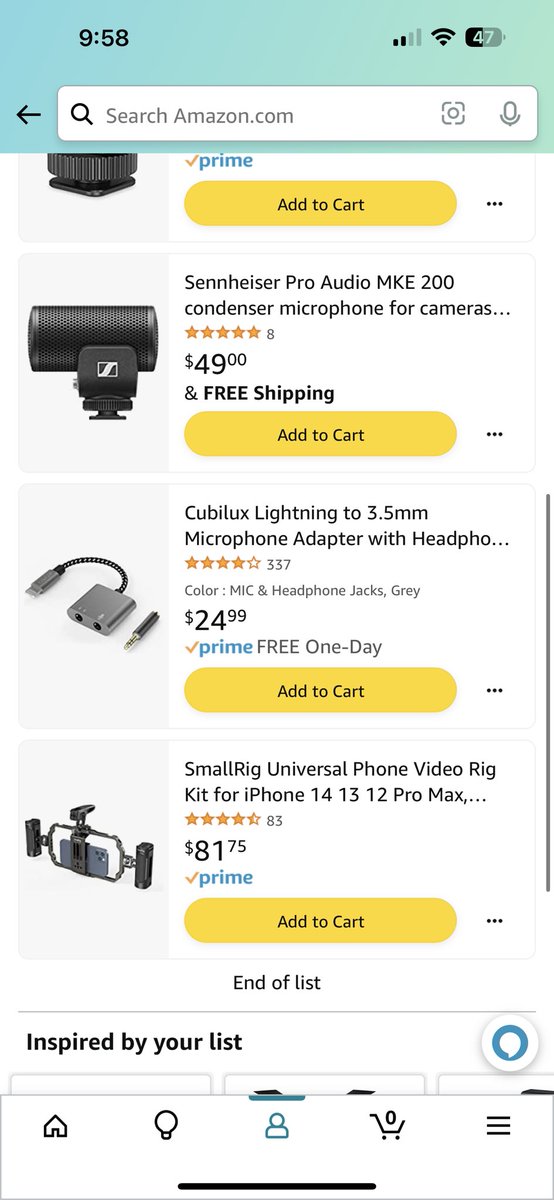A detailed and cleaned-up caption for the described image could be:

"A vertical rectangle displaying what appears to be a smartphone screen. At the very top, a turquoise box shows the time '9:58' in black. To the right, there is a Wi-Fi signal icon with two bars, followed by the Wi-Fi symbol, and a black square with '47' in white inside it. Below the turquoise space, a rectangular search bar contains a magnifying glass icon and the text 'search amazon.com,' along with a square icon featuring a circle and a microphone inside it. Outside of this box, on the left, there is a black arrow pointing left. 

Below the search bar, there are four images of products available for purchase. The first product appears to be some audio equipment displaying the Prime logo and has an orange 'Add to Cart' button, followed by three horizontal dots indicating additional options. The next three items follow a similar layout, each with a product image, some accompanying text, and an orange 'Add to Cart' button. 

At the bottom of the list, it says 'End of List,' followed by a bar indicating 'Inspired by your list,' next to which are several logos. Beneath all this is a square that likely represents further navigation or content."

This caption captures the detailed layout and content displayed on the apparent phone screen.